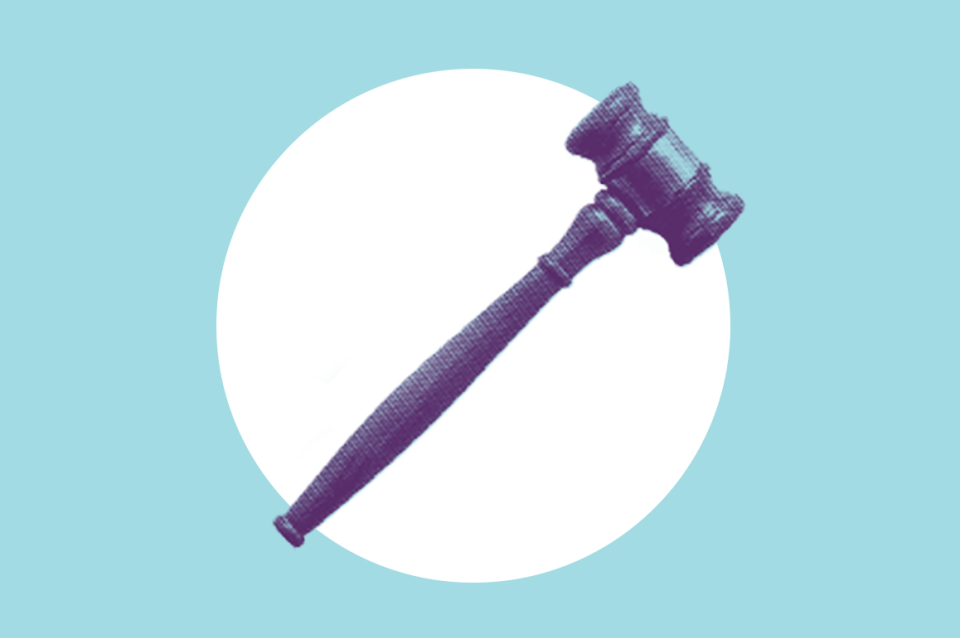The image depicts a stylized, pop art-inspired judge's gavel, rendered in a textured, newsprint or risograph-like quality. The gavel, with a purple hue and blue reflections, is positioned at a 45-degree angle atop a centrally located white circle. This circle contrasts against a pale aqua blue, almost sky-blue, background, giving it a clean and modern aesthetic. The gavel's handle is notably longer than a typical courtroom gavel. The detailed, somewhat blurry texture created by dots gives the gavel a distinctive, almost abstract appearance. This graphic design work, likely intended as an icon or banner, would be well-suited for a blog or article related to law.